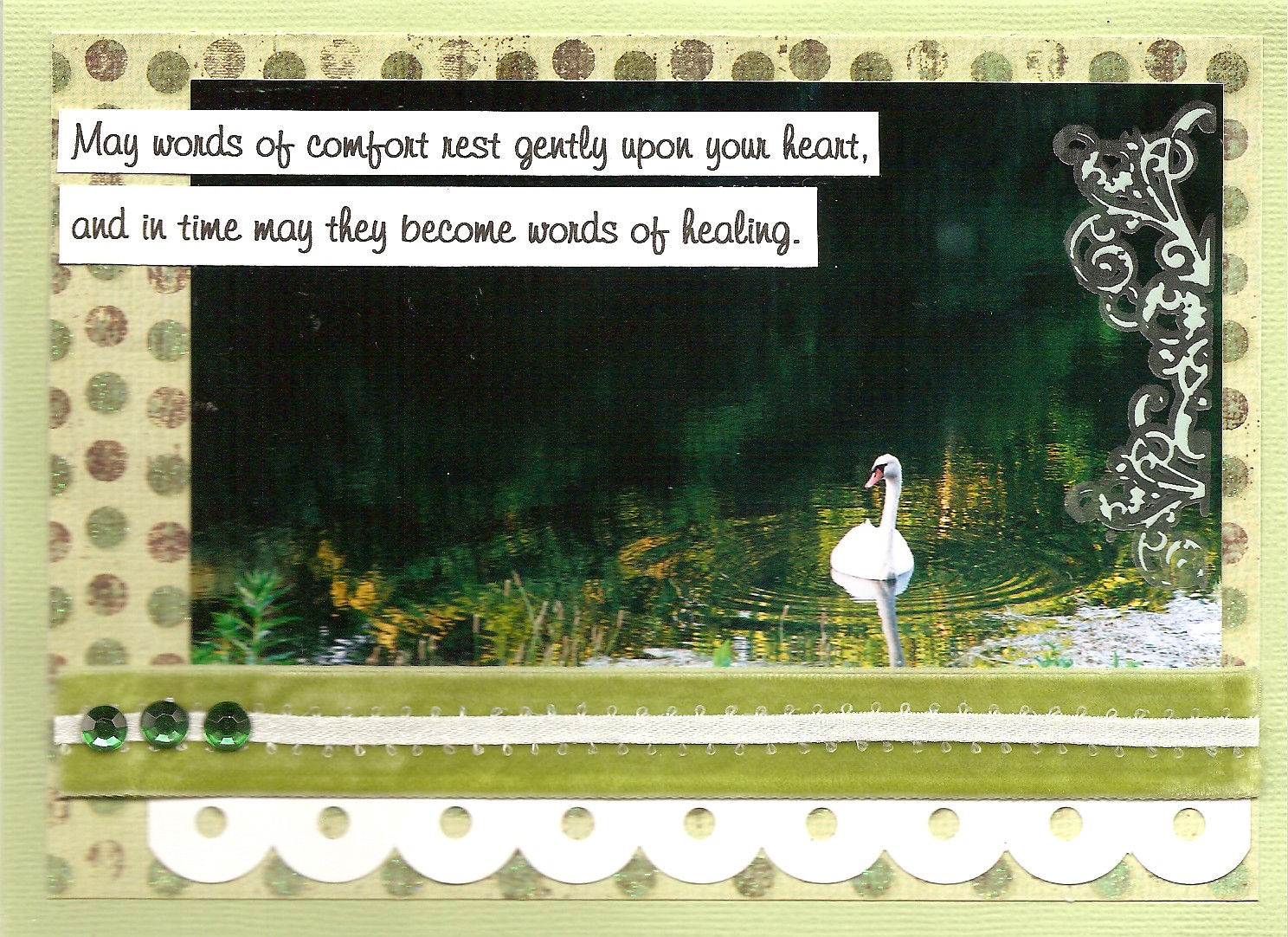The image features a serene photograph of a white swan with an orange beak, gracefully swimming in a greenish pond. The swan is positioned in the lower right corner of the picture. At the top, two stacked white banners with black script convey a heartfelt message: "may words of comfort rest gently upon your heart and in time may they become words of healing." Surrounding the photograph is a light green border, followed by a detailed area of polka dots, adorned with different pieces of material or cardstock. Adding a touch of elegance, a strip of velvet with three green jewels and an underlying strip of lace decorates the bottom of the image. The overall theme of the image, structured like a vintage sympathy letter, is enhanced by intricate scrollwork along the interior edge and a sophisticated beige postcard background with brown and light green polka dots.